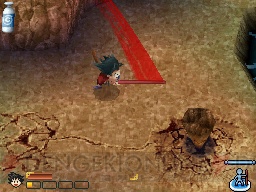In this rectangular digital scene, which appears to be a screenshot from a video game, the setting features a brown-colored floor or ground with a prominent crack running horizontally from the lower left corner to the center, where it stops at a diamond-shaped stone in a golden hue. At the heart of the image stands a character with long black hair styled to resemble spikes, giving it a porcupine-like appearance. The character has a brown body and is facing towards the crack. In the lower left corner, part of the character’s head is visible, along with rectangular shapes that could be elements of a scoring or progress tracking device, though no numerical values are discernible. A watermark that reads "Dengue Kean" diagonally spans across the image, subtly blending into the background.